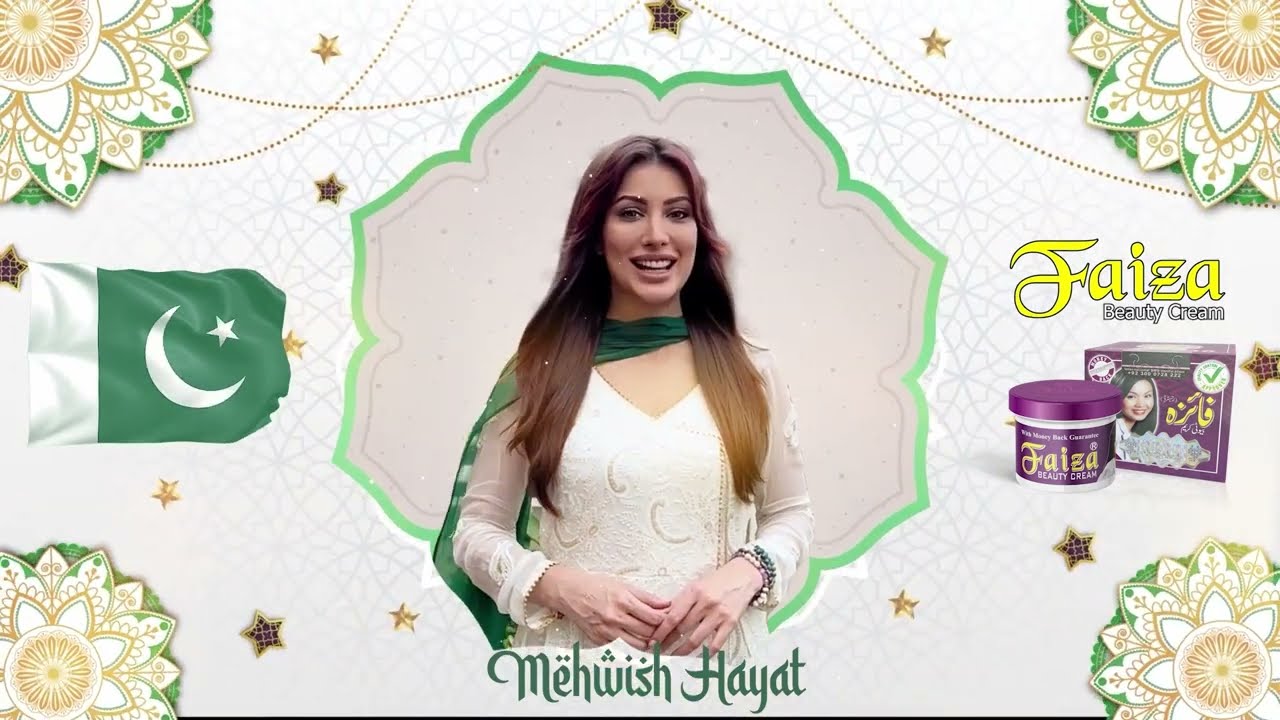The advertisement features an image with a clean, white background adorned with a subtle, abstract design of faint light gray lines. Each corner of the image showcases a floral motif with alternating patterns in white, gold, and green, including a white center, white leaves, and a combination of gold, green, and white outer leaves.

At the heart of the image is a striking, larger flower shape outlined in green, within which stands a beautiful woman with long, straight brown hair. She wears a green shawl draped over her shoulders and a white dress, complemented by bracelets on one wrist. The woman's serene smile and elegant attire enhance the overall aesthetic.

To the right of the woman, the name "Faiza" is prominently displayed in yellow letters, with "Beauty Cream" written directly below it. The product appears below this text, shown as a purple box alongside a matching purple container.

On the left side of the image, an Islamic flag is depicted, featuring a white rectangular stripe and a green field with a white crescent moon and star. The flag adds a cultural element to the advertisement, which is dedicated to promoting the Faiza Beauty Cream. The box of the cream also includes additional intricate details such as a check mark, beads, and possibly stars. Overall, the design effectively merges elegance and advertising, drawing focus to both the product and the graceful figure at the center.